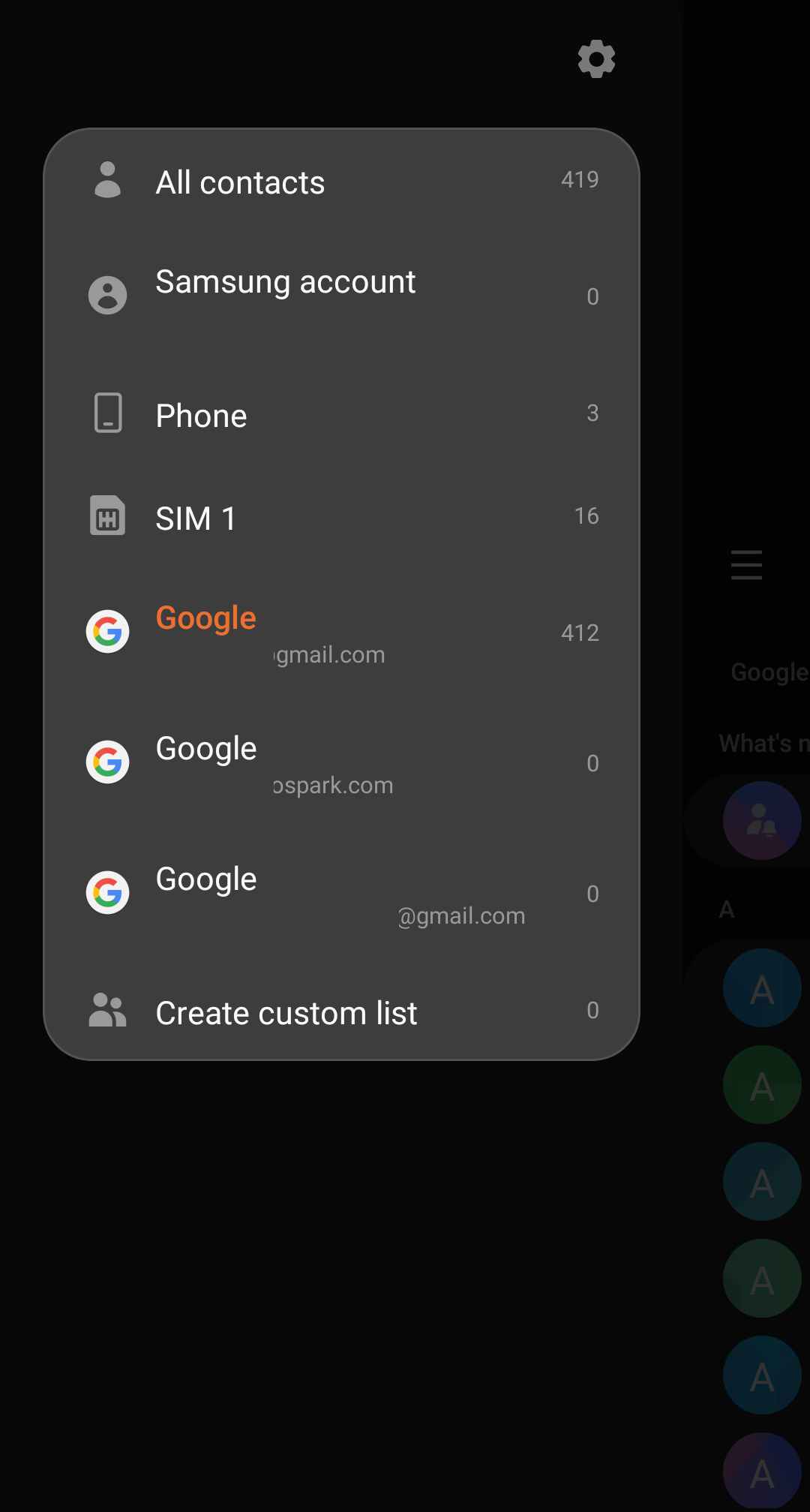This is a screenshot likely taken from a smartphone, displaying a preference or settings page. The background of this page is black, and a gear icon signifies the settings menu. Below this, there's a rectangular section that details the saved contacts across various accounts:

- **All Contacts**: 419
- **Samsung Account**: 0
- **Phone**: 3
- **SIM 1**: 16

There are also multiple Google accounts listed:
- The first Google account is partially obscured, ending in `gmail.com`, with 412 contacts.
- The second Google account is partially obscured, ending in `spark.com`, with 0 contacts.
- The third Google account, also partially obscured and ending in `gmail.com`, has 0 contacts.

At the bottom, there's an option to create a custom list, but currently, no custom lists have been saved.